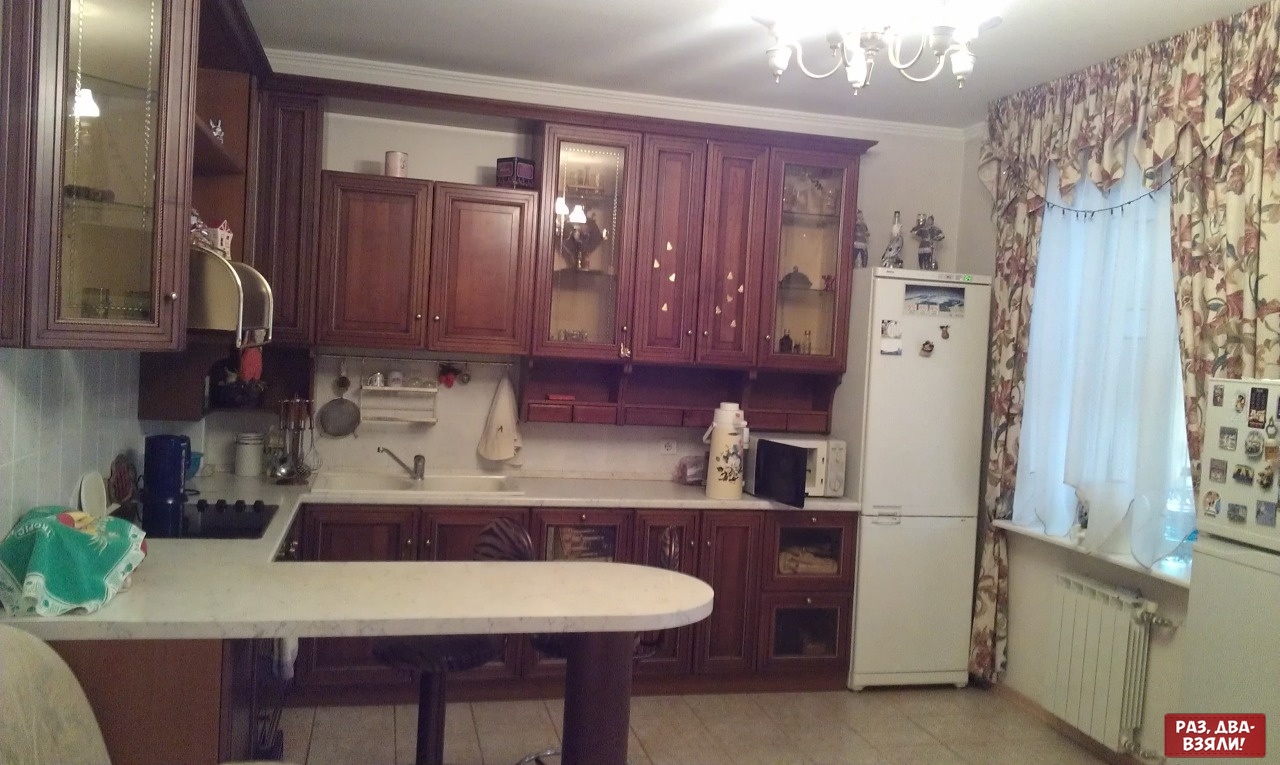This image showcases a vintage kitchen, characterized by its dated and somewhat antiquated style, evoking a sense of nostalgia reminiscent of the 1970s or 80s. The focal point of the kitchen is an island in the foreground, leading the eye to a cooktop on the left side of the kitchen. The countertops, likely granite or a similar material, create a squared C shape, wrapping around the left side and back wall, forming a cohesive workspace. Dark cherry wood cabinets, some with glass doors revealing their contents, provide ample storage. 

The kitchen features various appliances: a microwave with its door open, sitting on the counter next to a tall, skinny white refrigerator-freezer combo located in the right corner. A glass surface cooktop and a vent hood above it are prominently visible. A linoleum floor and white chandelier hanging from the ceiling add to the overall vintage aesthetic. 

On the far wall, a window dressed with sheer white curtains and a busy pattern of brown and green drapes illuminates the space. Below the window, an old-fashioned white coil heater stands out. 

The image also features some Russian or Cyrillic text in the bottom right corner against a red background with white letters, though the exact wording remains unreadable. Various kitchen items, including a tea kettle, utensils, and towels, contribute to the lived-in feel of this charmingly dated interior.